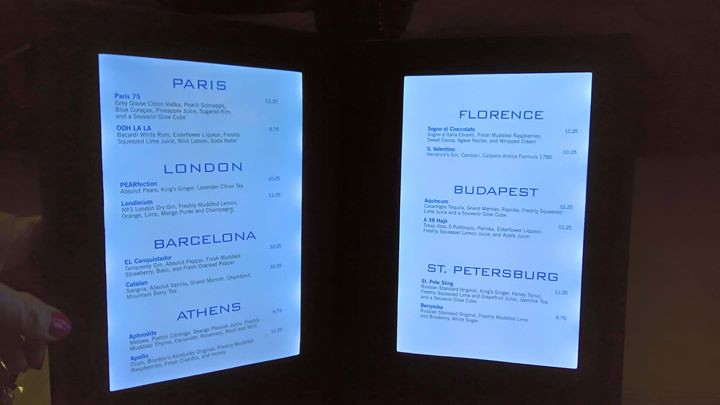In this dark and moody image, there are two illuminated white screens that display a sophisticated drink menu, creating a contrast against the black background. The left screen features a series of travel-inspired cocktail names with detailed descriptions and prices. Among these, there is "Paris 75," made with ingredients including Grey Goose, and another drink named "Ooh La La." Additional drinks listed include "London," "Purrfection," "Barcelona," "El Conquistador," "Catalina," "Athens," and "Aphrodite." Each drink name is followed by its ingredients and a price to its right.

The right screen, though slightly blurred, lists more exotic cocktails under headers such as "Florence," each accompanied by two types of drinks, and other sections labeled "Budapest" and "St. Petersburg." Despite the low visibility of the text, it is clear that these too have their ingredients and prices displayed. The black background behind the glowing screens offers no discernible details, emphasizing the focus on the enticing drink options.